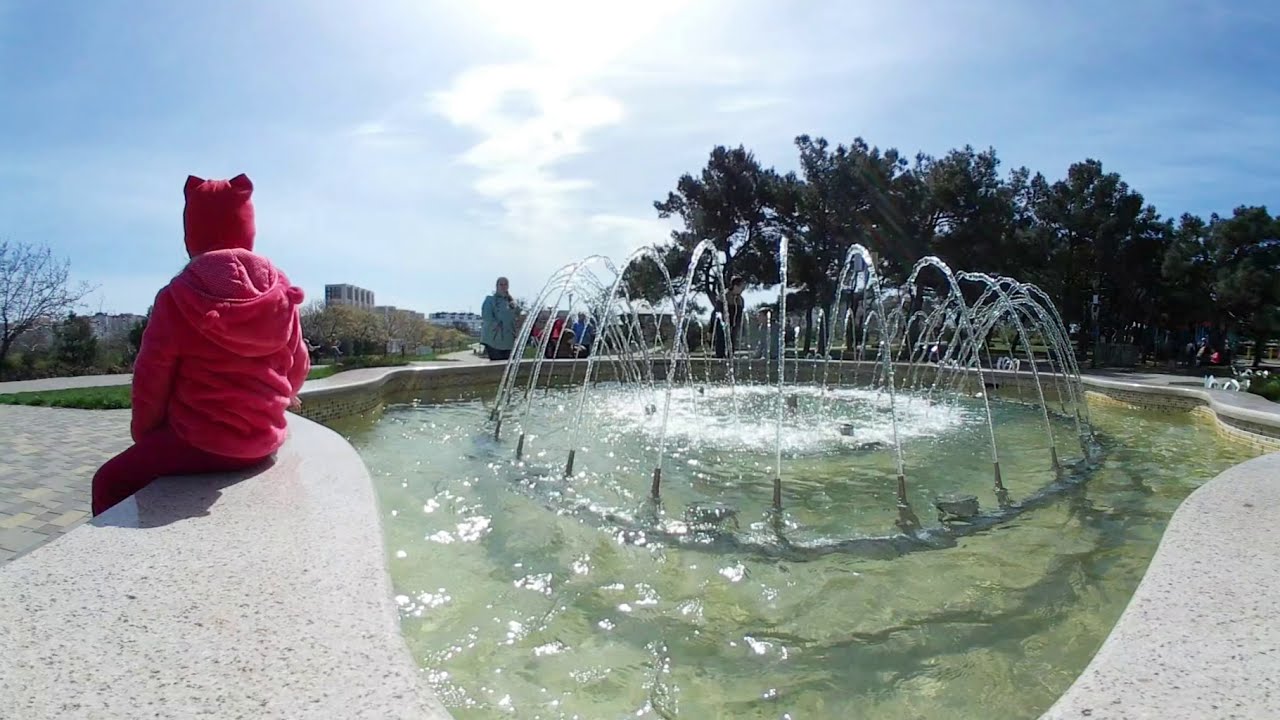In this outdoor daytime scene, a young child is positioned prominently in the center foreground, seated by the edge of an elliptical-shaped fountain at a park. The fountain features a ring of spouts that arc water into the center, creating a dynamic water display that captures a majority of the scene's focus. The child, identifiable by a red teddy bear hood with little ears and a matching pink, or possibly red, jacket and pants, faces away from the camera looking towards the background. This outfit detail, combined with the hat covering their whole head, suggests the child is a girl, though her face is not visible.

To the left of the child, another individual in a long white jacket below the waist also gazes towards the fountain and surrounding scene. Encircling the fountain is a sitting wall area, and beyond this are pathways, grass, and a mix of tall trees planted throughout the park. The background reveals a scattering of people and distant buildings, contributing to the lively atmosphere. The sun shines brightly from the top middle of the image, highlighting the clear day with a few clouds present in the sky.